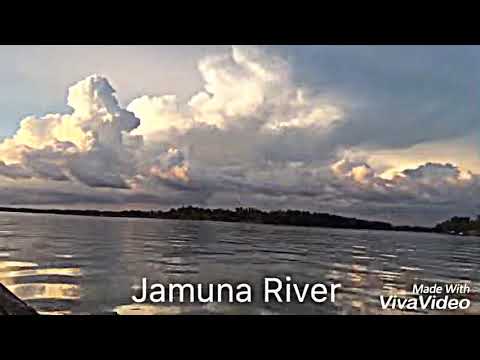This image titled "Jamuna River" (indicated by white text at the bottom) showcases a vibrant yet moody scene captured in lesser quality, likely due to it being a screenshot. The photo was created using Viva Video, as noted by italicized text in the bottom right corner. It depicts a river tinged with yellow sunlight reflecting off its surface, appearing dark and choppy with hues of brown and black. Above the river, the sky is dominated by a large structure of thick, fluffy clouds. The tops of these clouds are illuminated with a warm yellowish light, creating a stunning contrast to their dark, grayish bottoms. In the upper right corner, the sky is mostly covered with gray clouds, while a small patch of blue and sunlight peeks through on the upper left. The horizon features a mountainous range of trees and land in the distance, contributing to the photograph's dramatic atmosphere, all bathed in the diffuse light of an unseen sun.